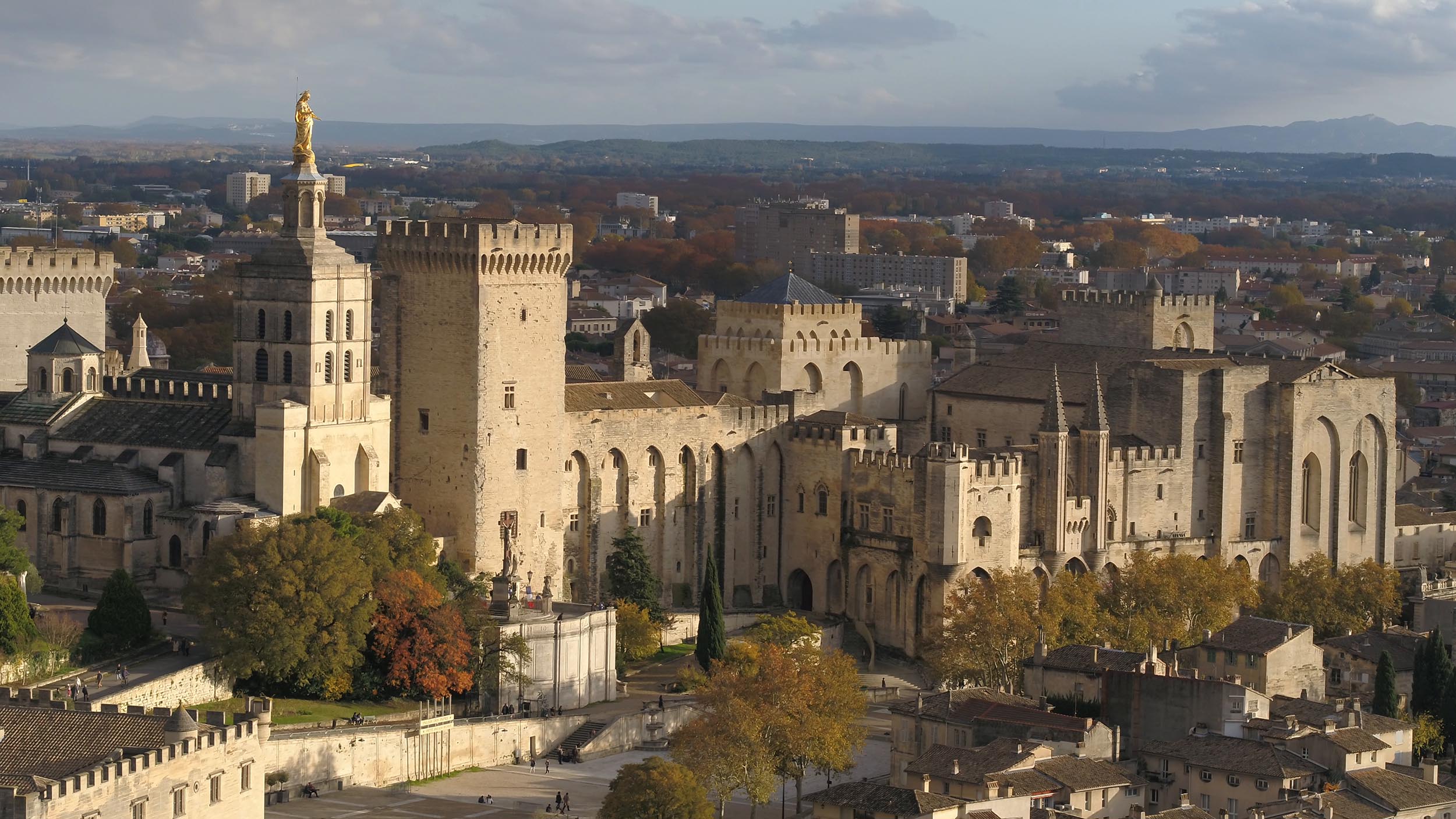This daytime photo captures an old-style stone fortress with a rugged, grayish façade, nestled amidst a blanket of dark green trees, indicative of late summer with touches of light brown. Dominating the top left tower is a gold statue, possibly a goddess, which stands as the tallest point of the structure. The fortress varies in height across its expanse, with some sections towering over others nearly twofold. From the distant vantage point of the photo, you can discern tiny people bustling in the streets below. Modern buildings with brown roofs cluster towards the bottom right, their stone-like architecture blending seamlessly with the historic landscape. The sky above is heavy with dark, brooding clouds interspersed with lighter shades. In the top right corner, the faint outline of distant mountains overlays the horizon, adding to the depth of the scene. Hints of early autumn appear in the foliage below, with patches of trees beginning to change color.